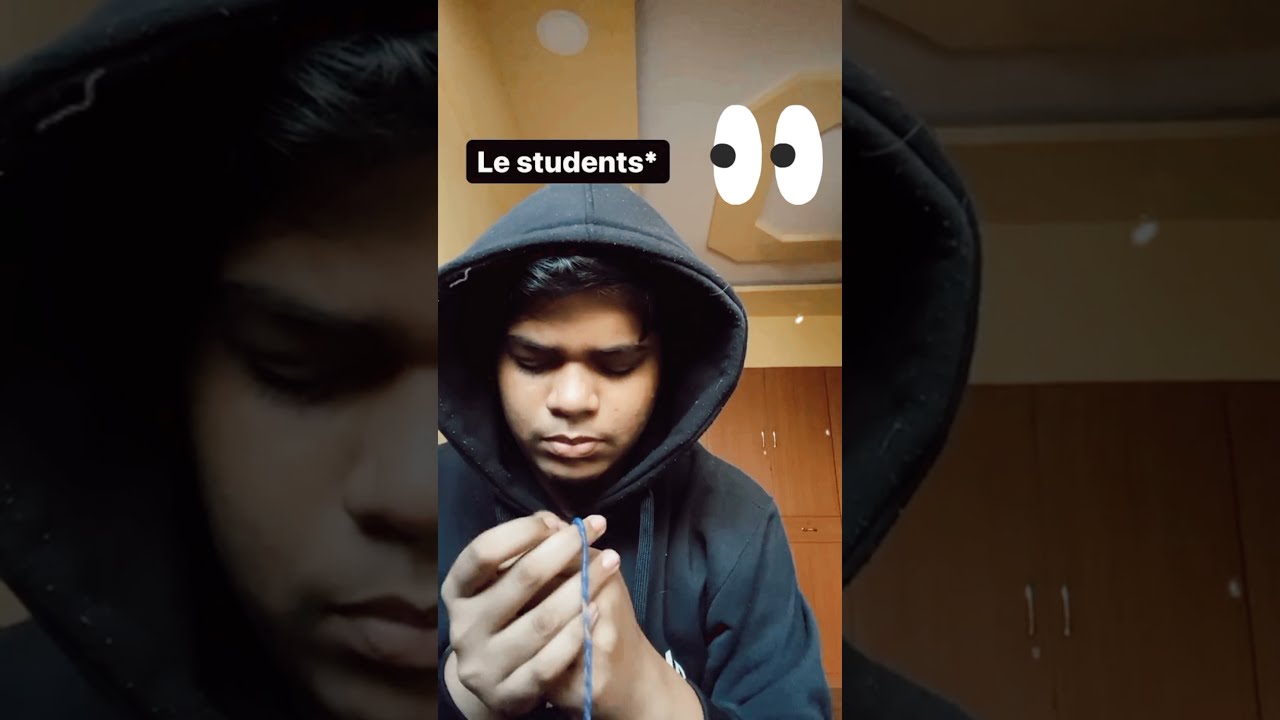The image appears to be a screenshot from a social media post, possibly a video or reel on platforms like TikTok or Instagram. It features a young man, possibly of Pakistani descent, sitting in what looks like a locker room with brown lockers behind him. He is wearing a black hoodie with the hood up, partially covering his black hair and eyebrows, and his mouth is closed. The man is intently gazing at something obscured by his hands, from which a blue string emerges and remains visible in front of his fingers. The photograph is taken from a slightly elevated angle, showing a ceiling that transitions from a yellow area to a white segment adorned with cream molding and pot lights. Above the man, in a black-bordered caption, the text "Le Students*" is displayed in white, accompanied by an emoji of two shifty eyes to the right. Additionally, there are darker, close-up overlays of the man’s face on either side of the main image, creating a bordered effect.